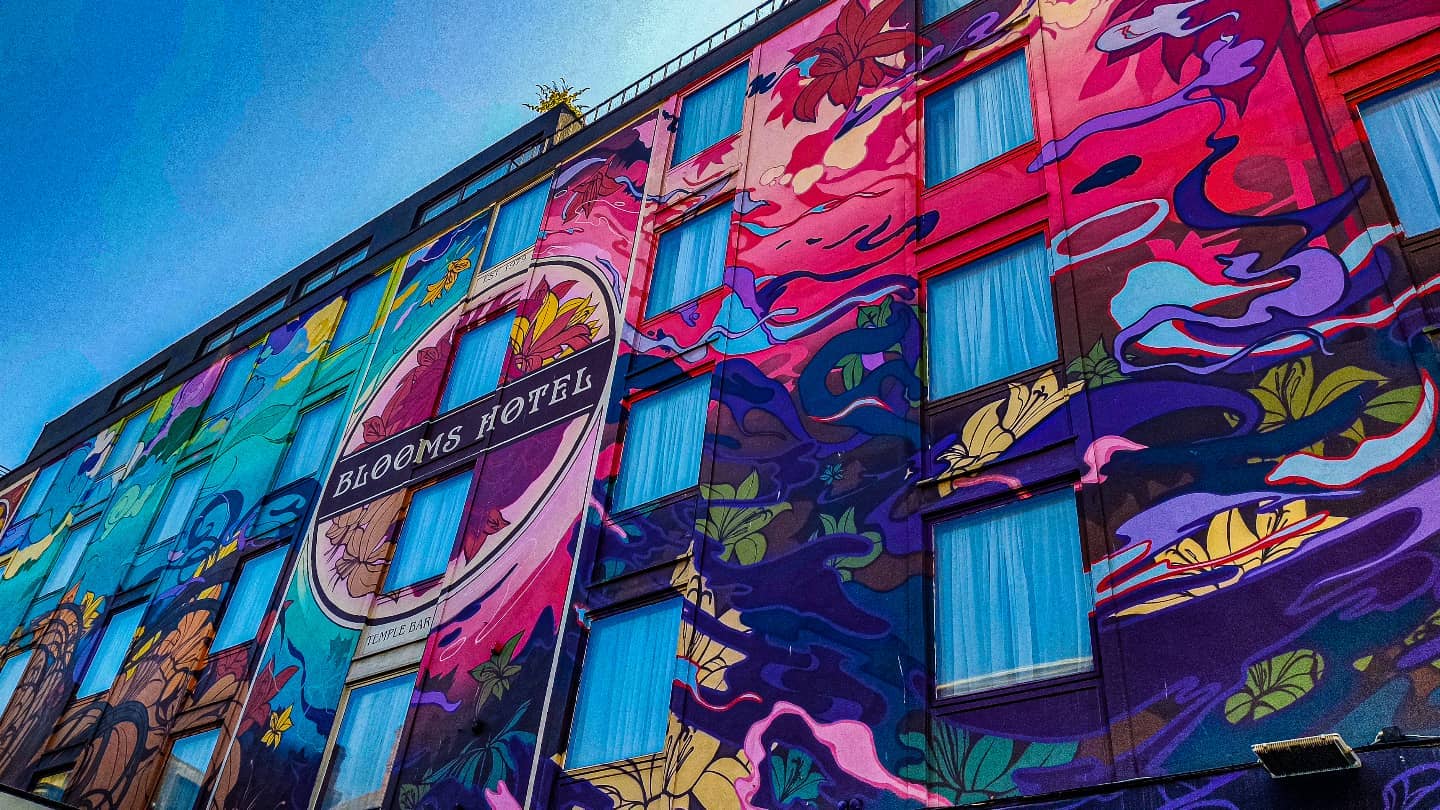The photograph captures the vibrant front facade of Blooms Hotel, viewed from a ground-level perspective, looking up towards the rooftop. The building spans four stories, each floor adorned with numerous windows, all featuring closed light blue curtains. The exterior of the hotel is strikingly colorful and vividly painted, with no visible brick texture, suggesting a flat surface. The artistic decoration covers the entire surface except for the windows and centers around a bold floral motif. The top right bursts with splashes of pink, the bottom right radiates with yellow and purple hues, the top left displays a blend of blue and turquoise, while the bottom left showcases a mix of brown and black adorned with gold flowers. The design incorporates an almost cartoonish style featuring elements like lily pads and flowing patterns, evoking a dynamic sense of movement as if water or smoke intertwines among the flowers. In the middle of this lively canvas, encircled prominently, are the words "Blooms Hotel." At the very top, an additional floor on the rooftop can be seen, possibly with some plant life, enhancing the floral and somewhat tropical theme of the hotel's facade.